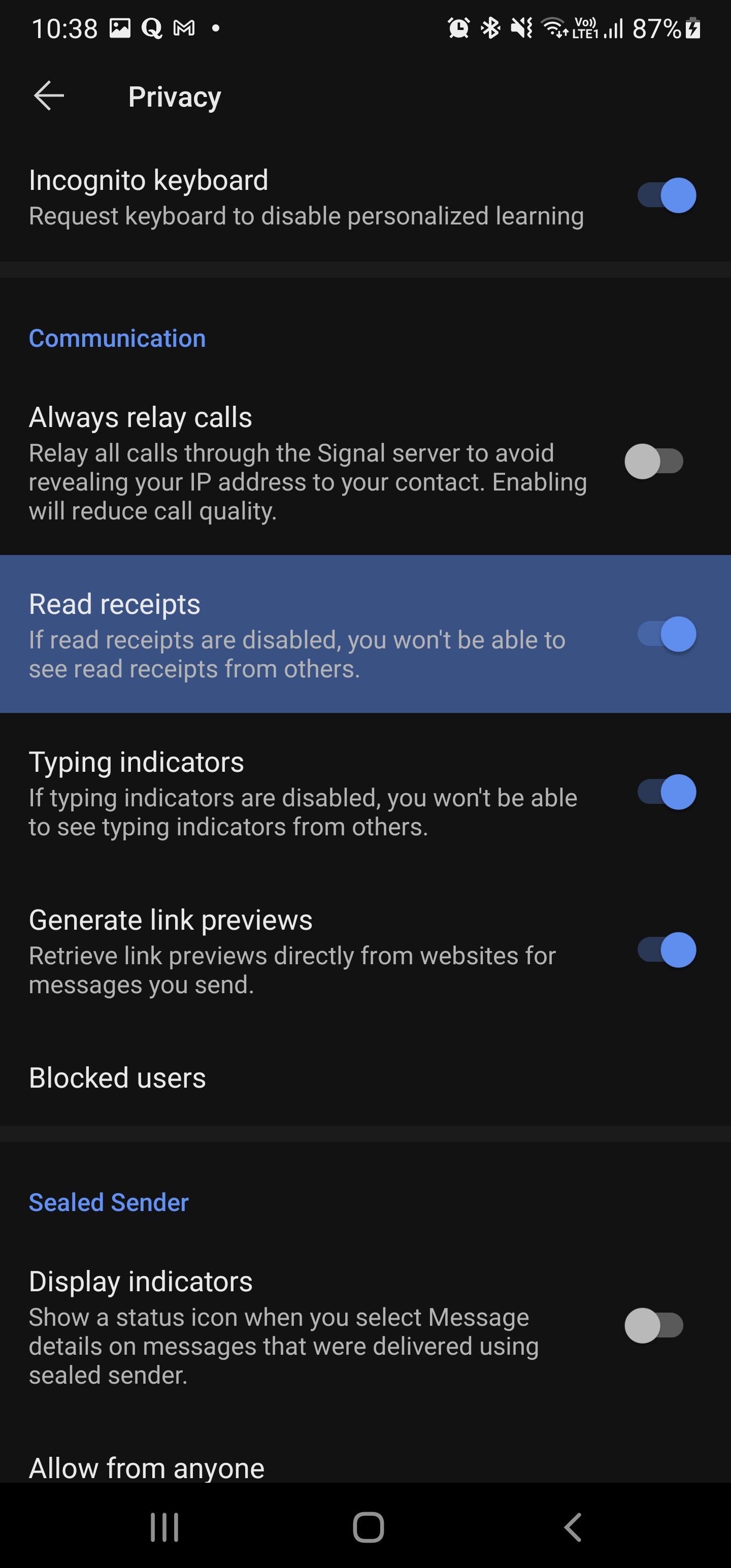The screenshot depicts a smartphone screen with a black background. At the upper left-hand corner in white font, the time is displayed as 10:38. On the upper right-hand side, a battery icon is visible, which is white with a black lightning bolt indicating that the phone is being charged. The current battery level is 87%.

Beneath the header, towards the left side, the word "Privacy" is written in white font, accompanied by a left-pointing arrow. Below this, "Incognito Keyboard" is listed with a description stating, "Request keyboard to disable personalized learning," and this option is chosen, indicated by a blue dot on the right side.

Further down, "Communication" is written in blue font. Underneath, in white font, "Always Relay Calls" is displayed with the note, "Relay all calls to the signal server to avoid revealing your IP address to your contact. Enabling will reduce call quality," and this option is not selected. This section is highlighted in a purplish-blue strip with white font, reading: "Read Receipts: If read receipts are disabled, you won't be able to see read receipts from others."

Returning to the black background, additional options are listed:
- "Typing Indicators"
- "Generate Link Previews"
- "Blocked Users"

In blue font, "Sealed Sender" appears, followed by "Display Indicators" in white font with the option "Allow from Anyone" specified below it. 

At the bottom of the page, the lower border contains a white circle on the left, three lines within the circle, and a small arrow pointing to the left on the right side.